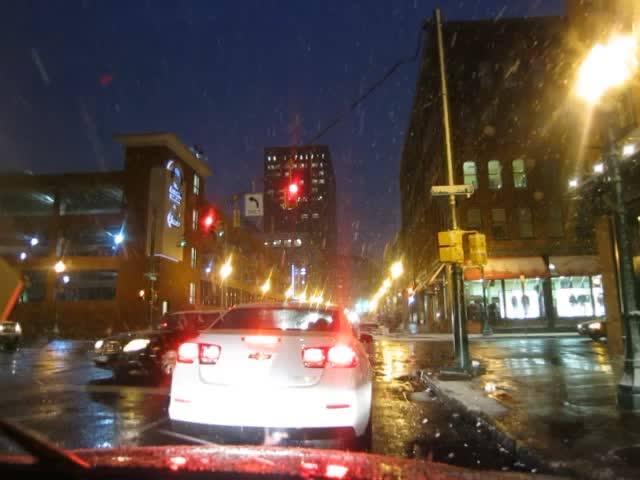This photograph, taken from within a vehicle, showcases a bustling urban street scene at night. Centered in the image is the back of a white Chevrolet sedan with its glowing taillights, stopped at a red traffic light. The wet streets, reflecting the multicolored city lights, indicate a recent mix of rain and melting snow. Another dark-colored car is making a left turn at the intersection in front of the Chevrolet. The scene is set against a backdrop of tall buildings, suggesting a commercial district, with some windows brightly lit. To the right, there's a brown building featuring a storefront with a red awning sprinkled with snow. A parking garage is noticeable to the left, and further illumination comes from street and stop lights. The sky above is a deep blue-purple, emphasizing the nighttime setting.